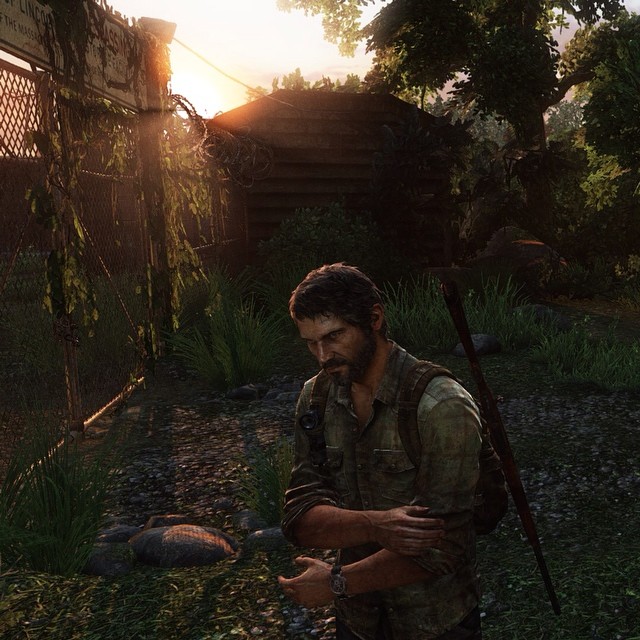In this screen grab from a post-apocalyptic video game resembling The Last of Us or Fallout, the image centers on a rugged man in the foreground. He is clutching his left arm as if injured or exhausted. Dressed in traditional apocalypse attire, he sports a weathered khaki button-down shirt, disheveled and dirty, paired with dark jeans. A rifle is slung over his shoulder, and a worn backpack is strapped to his back. His unkempt hair and scruffy beard suggest he hasn't bathed in a while. Behind him, an overgrown fence sets the boundary for a dense, forest-like jungle scene, with an old wooden shack partially visible in the background. The ground beneath his feet is a mix of overgrown gravel and scattered stones, emphasizing the desolate, neglected environment.